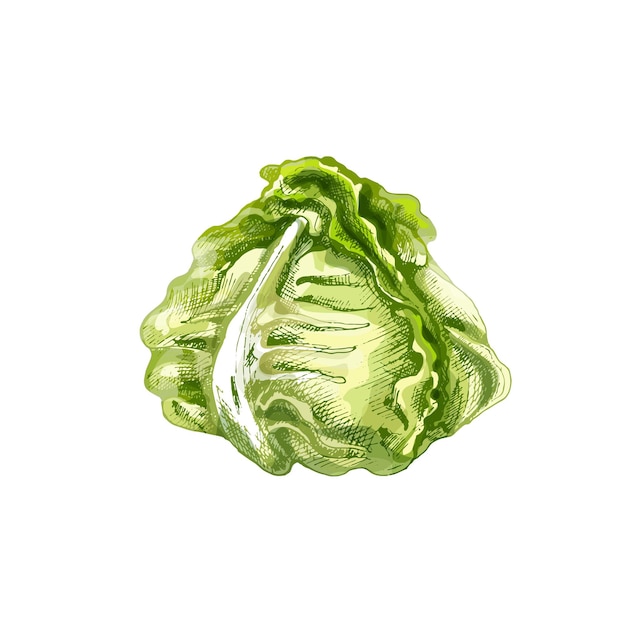This image showcases an artistic drawing of a head of iceberg lettuce against a solid white background. The illustration employs a combination of watercolor and pen-and-ink techniques, lending it an abstract yet detailed appearance. Multiple shades of green are used to capture the varying hues of the lettuce, from dark green ruffles at the top to lighter greens and almost white near the ribbing. The texture of the leaves is intricately depicted with cross-hatch shading, particularly noticeable in the darker green areas and the white ribbing. The curly leaves, positioned facing upwards, display precise detailing with little lines and cross-hatches, enhancing the drawing's depth and realism.